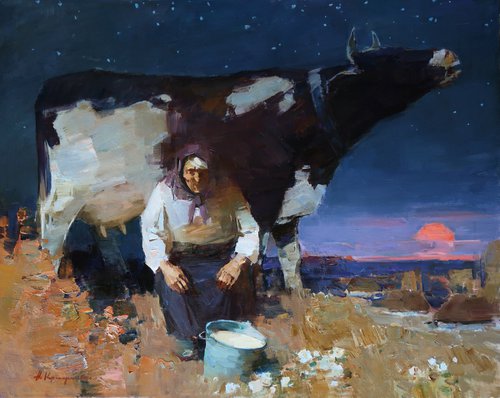This watercolor painting beautifully captures a tranquil farming scene at sundown. The focal point is a black and white cow, its head raised in what appears to be a moo. In front of the cow sits a woman, adorned in a purple headpiece, a long-sleeve white shirt, and a dark blue skirt. She is milking the cow into a silver bucket brimming with milk. Nestled within the tall grasses, interspersed with white and green flowers, they sit on barren, brown-toned ground with scattered brown and tan rocks visible in the distance to the right. Above them, the sky transitions from a vivid blue to a darker blue as stars begin to twinkle. An orange half-sphere sun sets over the water, casting a serene glow and bringing the day's end to this pastoral landscape.